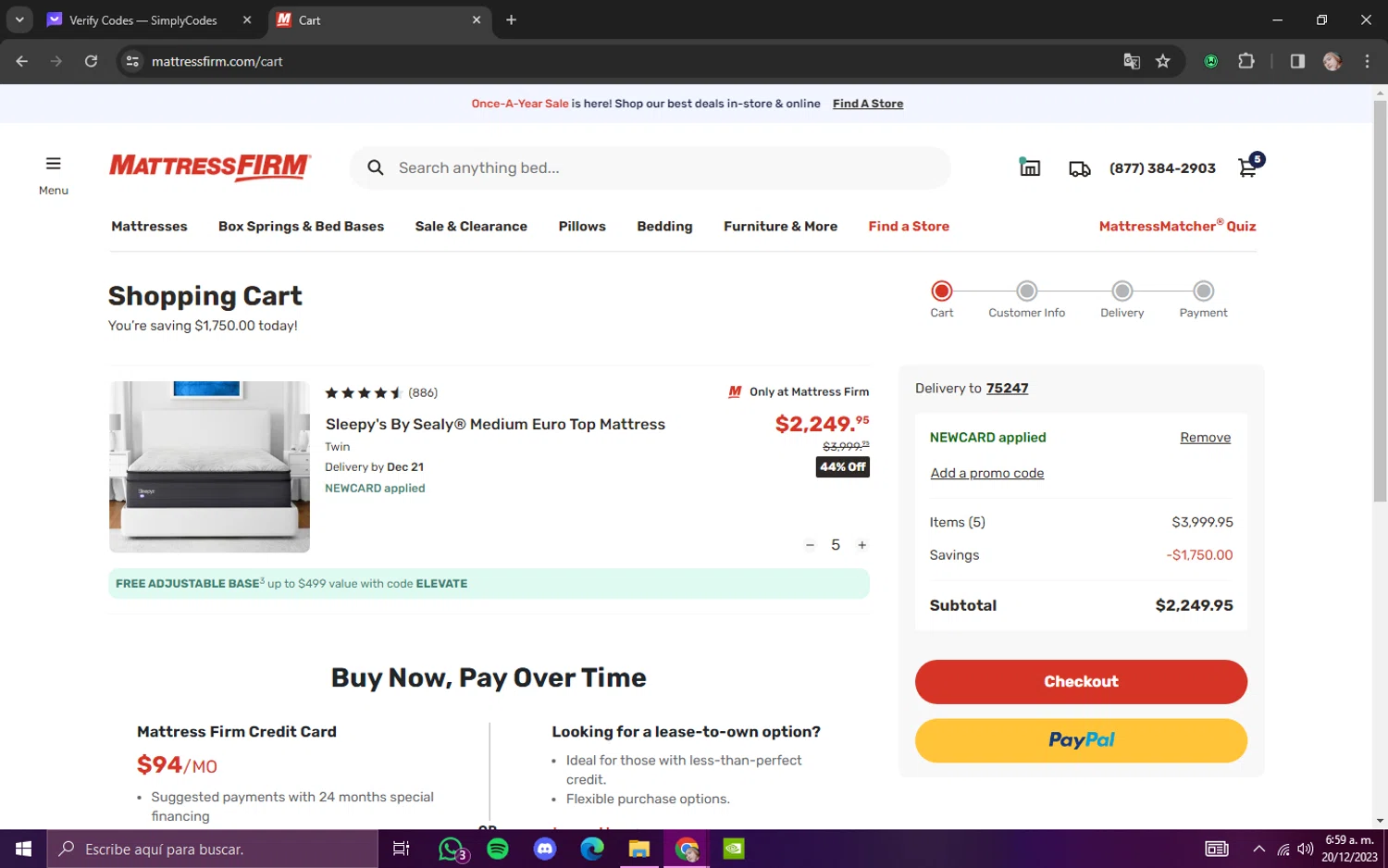This image is a detailed screenshot of a shopping cart page from the Mattress Firm website. At the very top, there is a black navigation bar extending the full width of the screen, featuring two tabs: one labeled "Verify Codes-Simply Codes" and another with an orange icon displaying an 'M' and the text "CART," which is currently selected. The URL in the address bar reads "MattressFirm.com/CART."

The main section of the webpage has a clean white background. Prominently displayed in orange text is the phrase "Once a Year Sale," followed by black text stating, "Here, Shop Our Best Deals In-Store and Online." Below this text, there is a clickable option titled "Find a Store." The page also showcases a red Mattress Firm logo adjacent to a search bar labeled "Search Anything Bed..." On the top right corner of the screen, a phone number (877-384-2903) is visible, along with a shopping cart icon.

The website menu lists the options "Mattresses," "Box Springs and Bed Bases," "Sale and Clearance," "Pillows," "Bedding," "Furniture and More,” "Find a Store," and the "Mattress Matcher Quiz.” 

Below the menu, it indicates that the user is viewing their shopping cart and proudly states, "You're Saving $1,750 Today." The featured product is shown with an image of a mattress set on a bed base. The product is identified as a "Sleepies by Sealy Medium Euro Top Mattress," boasting a rating of 4.5 stars from 886 reviews, exclusively available at Mattress Firm. The listed price is $2,249.95, which reflects a 44% discount. 

A green bar beneath the product image advertises a "Free Adjustable Base up to $499 value with code ELEVATE." Additional financing information is provided, including an option to "Buy Now, Pay Over Time" using the Mattress Firm Credit Card with monthly payments of $94. There is also mention of a lease-to-own option.

On the right-hand side of the screen, a summary column includes delivery to the zip code 75247, a "New Card Applied" status, a section for adding a promo code, and an order summary listing 5 items totaling $3,999.95 with savings of $1,750, bringing the subtotal to $2,249.95. Finally, there are red and yellow ovals for "Checkout" and "PayPal" payment options, respectively.